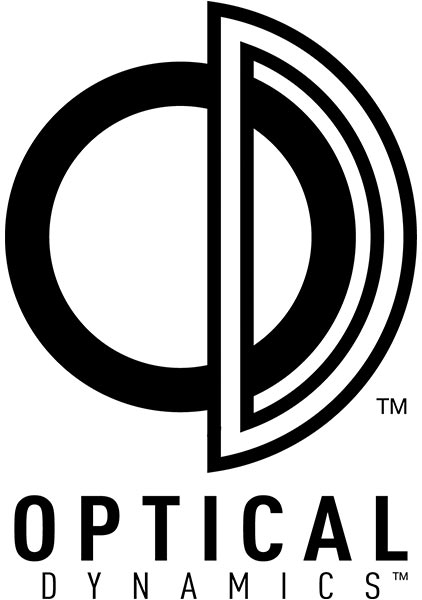This image is a detailed close-up of the Optical Dynamics logo, displayed on a white background. At the center is a thick, black ring that is intersected on the right side by a large, capital 'D.' The 'D' is black and outlined in white. Adjacent to the lower right of the 'D,' the trademark symbol 'TM' appears in black. Below the ring, the word 'OPTICAL' is prominently featured in large, solid black, bold, uppercase letters. Beneath 'OPTICAL,' the word 'DYNAMICS' follows in smaller, black, uppercase letters, with wider spacing between the letters compared to 'OPTICAL.' The trademark symbol 'TM' is also positioned after 'DYNAMICS.' The overall design is simple yet striking, utilizing bold black on a clean white background.